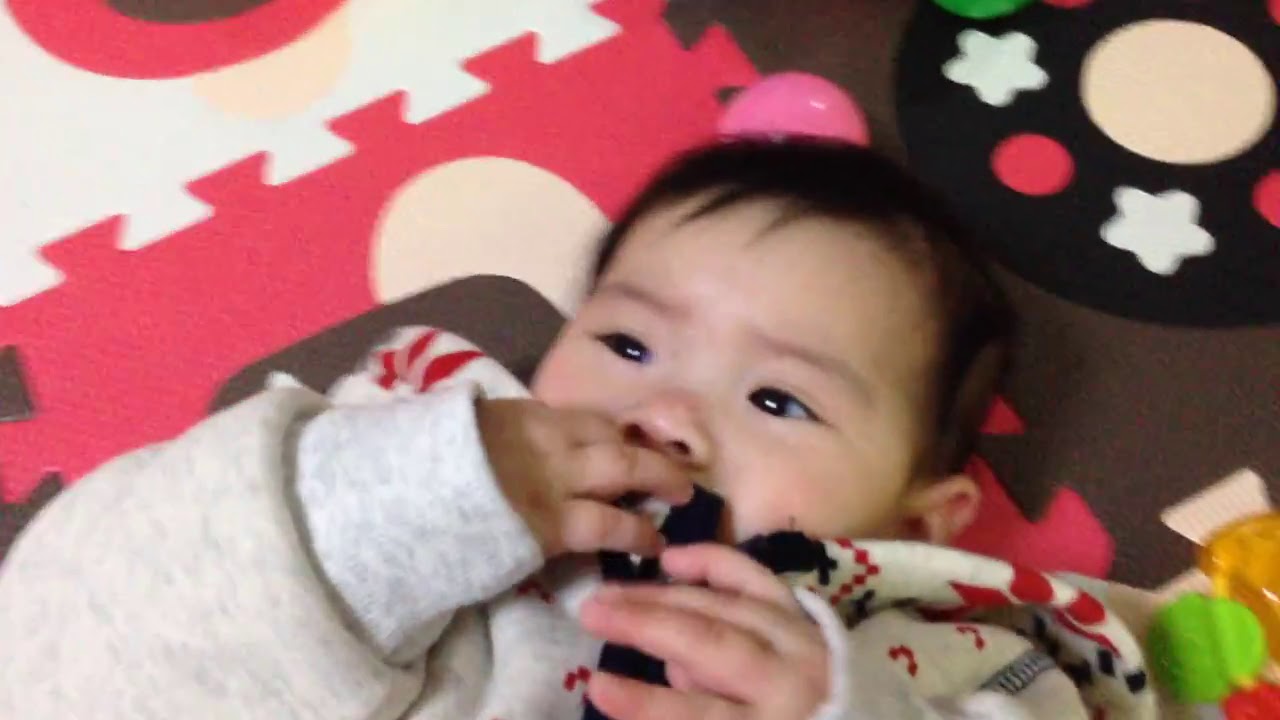The image features a baby of Asian descent, sitting and slightly leaning to the top right. The baby, with short brown hair and thin, straight eyebrows, is dressed in a grayish sweater and seems to be chewing on a small black object. The left hand is holding this object against the mouth, while the right hand grasps its end. The baby is lying on a pink and white mat that has a puzzle-like pattern. A cozy white blanket with red and possibly black designs is wrapped around the baby. Nearby, there's a colorful baby toy in yellow, green, and red, possibly a dangling rattle. The background also includes a carpet with a circular design featuring white stars, pink dots, and some green dots embroidered within it.